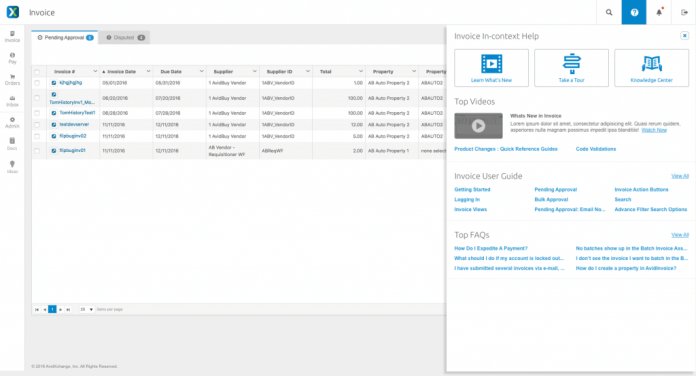The screen displays a web page titled "Invoice," predominantly in white with gray and blue text. On the left side of the page, there is a vertical menu with various tabs, although they are too small and blurry to distinguish clearly. This menu appears to list different options and includes two main tabs.

The top right corner of the web page features several icons: a magnifying glass, a question mark, a bell, and another unidentified icon. The question mark icon has been clicked, opening a tab labeled "Context Help." This section includes three clickable options under the "Invoice" heading. Below that, there is a section titled "Top Videos," with a list of clickable blue links, such as "Invoice User Guide" and "Top FAQs," which presumably provide further information.

Despite the overall layout and available options, the small and blurry text makes it difficult to read most of the details. The web page also offers a feature to "Take a Tour" at the top.